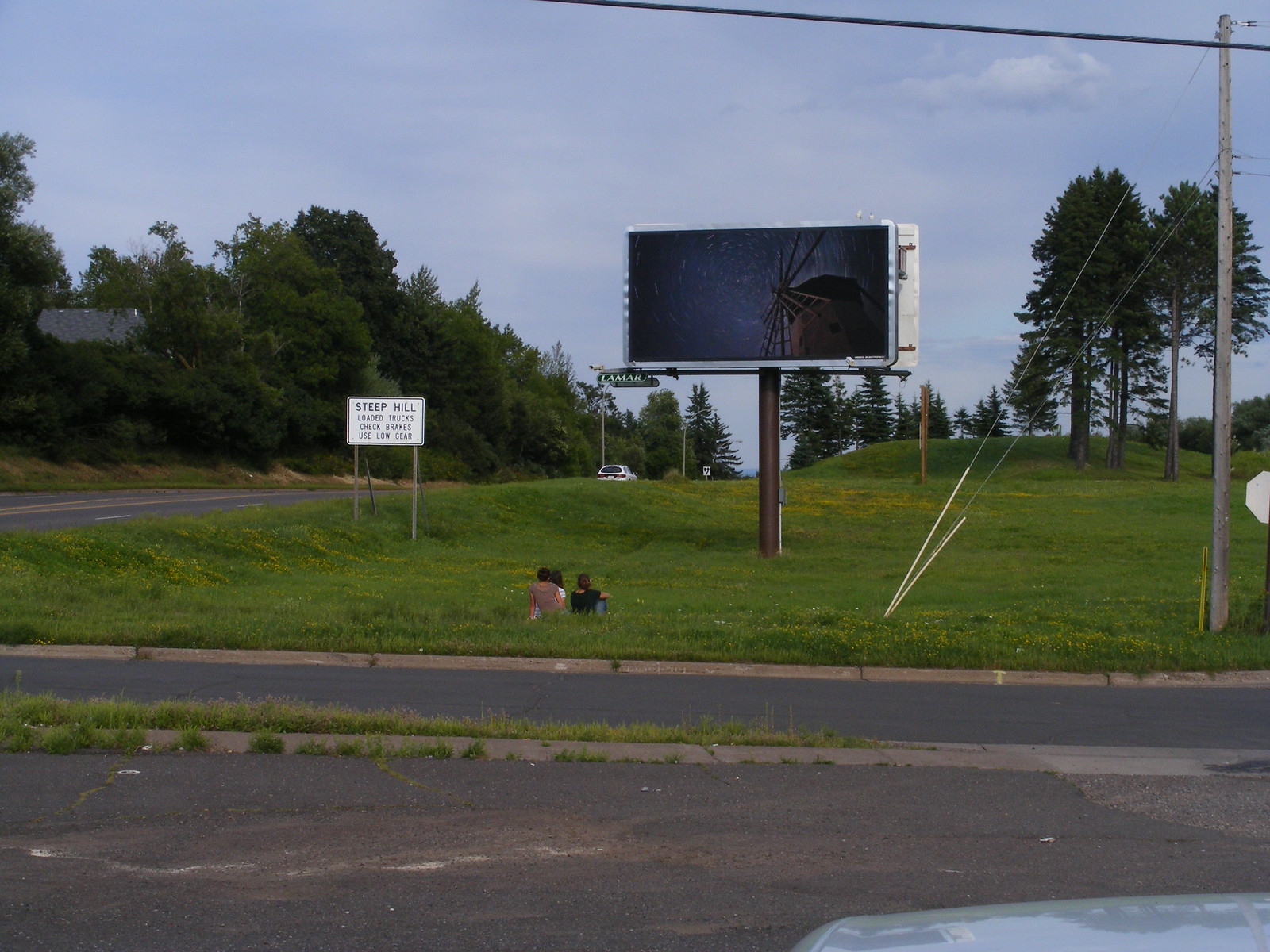A vibrant outdoor scene features a busy landscape dominated by a light blue sky adorned with patches of gray clouds over a lush, green hill. At the forefront, a bee hovers near the vivid, crisp green leaves of a nearby tree, while an expanse of thick, verdant trees stretches across the background. Prominently, a digital billboard displaying a video of a windmill stands out amidst the greenery. To the left, a road winds into the distance, accompanied by a white fence that contrasts sharply against the foliage. A white sign with black lettering reading "Steep Hill" is also visible on the left side. On the far right, a tall pole extends into the sky, its attached line anchoring it firmly into the ground. The asphalt road in the backdrop is cracked and leads to a gray sidewalk, where a solitary figure sits, captivated by the digital display on the billboard.